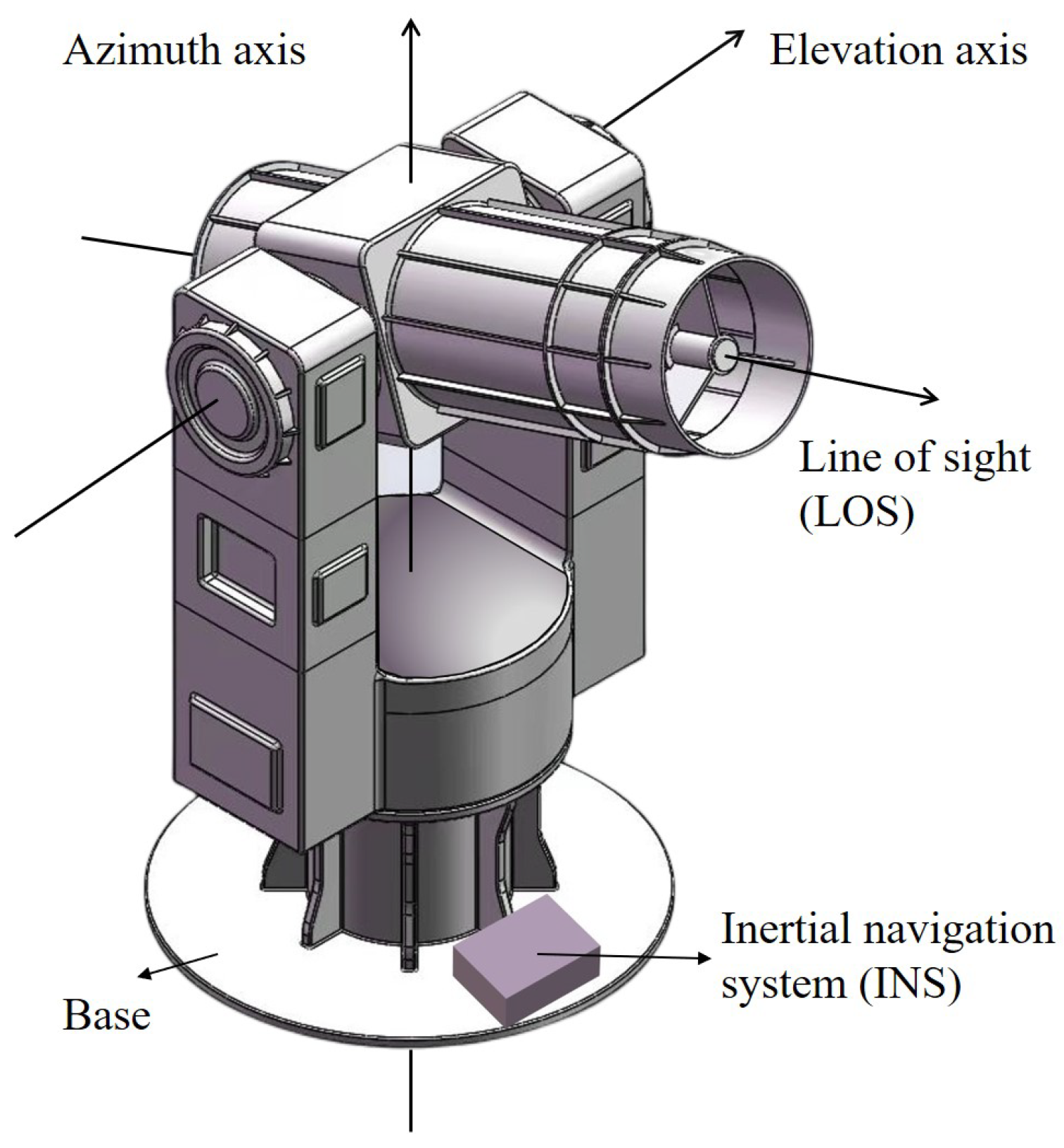This illustration appears to depict a sophisticated navigation camera or sensor system, likely from a technical or educational textbook. The main structure stands on a round white base marked "BASE," which supports the entire apparatus. Elevated upon the base is a metallic, cylindrical mechanism with several labels indicating key functional components. 

At the bottom, adjacent to the base, there is a label for the "Inertial Navigation System" (INS), which suggests the device relies on internal measurements to navigate or maintain balance. A small box also labeled "Inertial Navigation System INS" sits on the ground near the base. Above this section, on the left side, an arrow points directly upwards labeled "Azimuth Axis," while on the right side, another arrow points diagonally labeled "Elevation Axis." Both axes likely relate to the rotational capabilities of the device, enabling it to pivot and adjust its orientation.

Prominently, the image shows a cylindrical section with a protruding lens or sensor at the front, signified by a label "Line of Sight" (LOS) with an arrow pointing straight outwards. This feature indicates the primary direction in which the device views or measures.

The structure includes a set of silver, rectangular boxes flanking the main cylinder, which contain various knobs and buttons, potentially for adjustments or calibrations. The shading of these components varies, with lavender on one side and silver on the other, adding depth and a tactile quality to the overall design.

Additionally, part of the image appears to be incomplete, with some arrows and labels only partially visible, suggesting that the full context may include further annotations not present in this segment. Overall, this complex, labeled diagram functions to explain the various components and axes involved in the operation of the inertial navigation and line of sight systems.